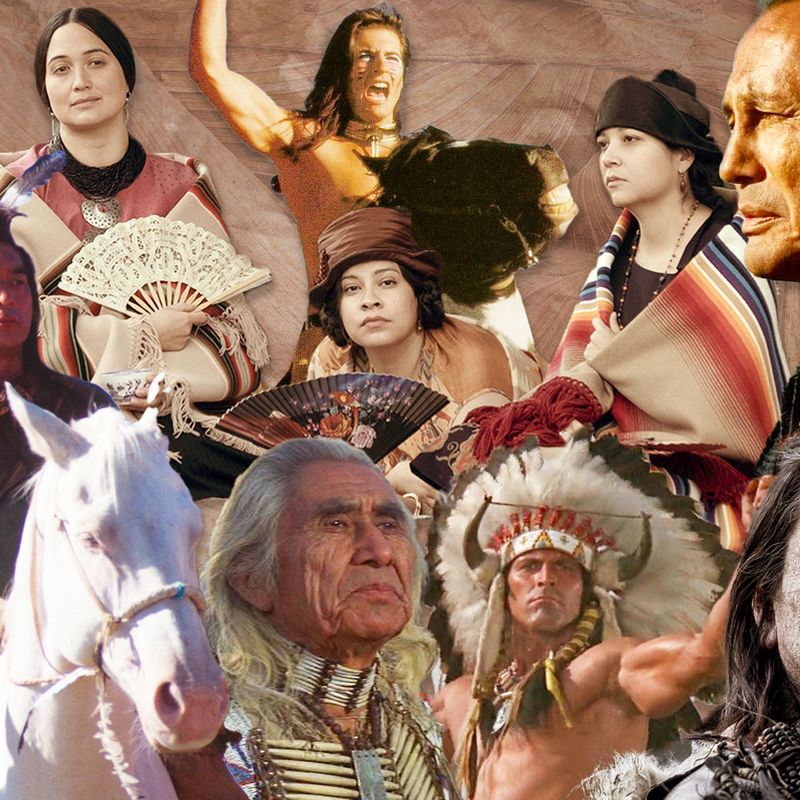The image is a vibrant collage featuring various Native American characters and actors from different films, meticulously cut out and pasted together against a clay-colored red background. On the far left, there's a graceful white horse beside an elderly Native American man with long, reddish-white hair and a deeply wrinkled, tan face. Adjacent to him, another character stands in the background, adorned in a large, white and black headdress. To the right, part of another person is visible, though their face is cut off.

Above, there is a row of about six distinct Native American figures, each from different movies, depicting different hues and varying image qualities. There’s a woman in the upper left corner, dressed in a Native American outfit with brown hair, a necklace, and an orange shirt covered by a tan blanket. Near her stands a man with a feather in his hair, reinforcing the cultural imagery.

The central part of the collage showcases a character on a horse with their right arm raised and makeup under their eyes, giving a sense of motion and intensity. Below this figure, a woman wears a brown hat. Next to her, an old chief dons a white chest plate, possibly made of bones, and has something white around his neck. To the right is a younger Native American man, shirtless and wearing an elaborate headdress with horns and white fuzz.

Overall, the collage captures a diverse array of Native American portrayals, blending timeless imagery with a palpable sense of historical and cinematic reverence.